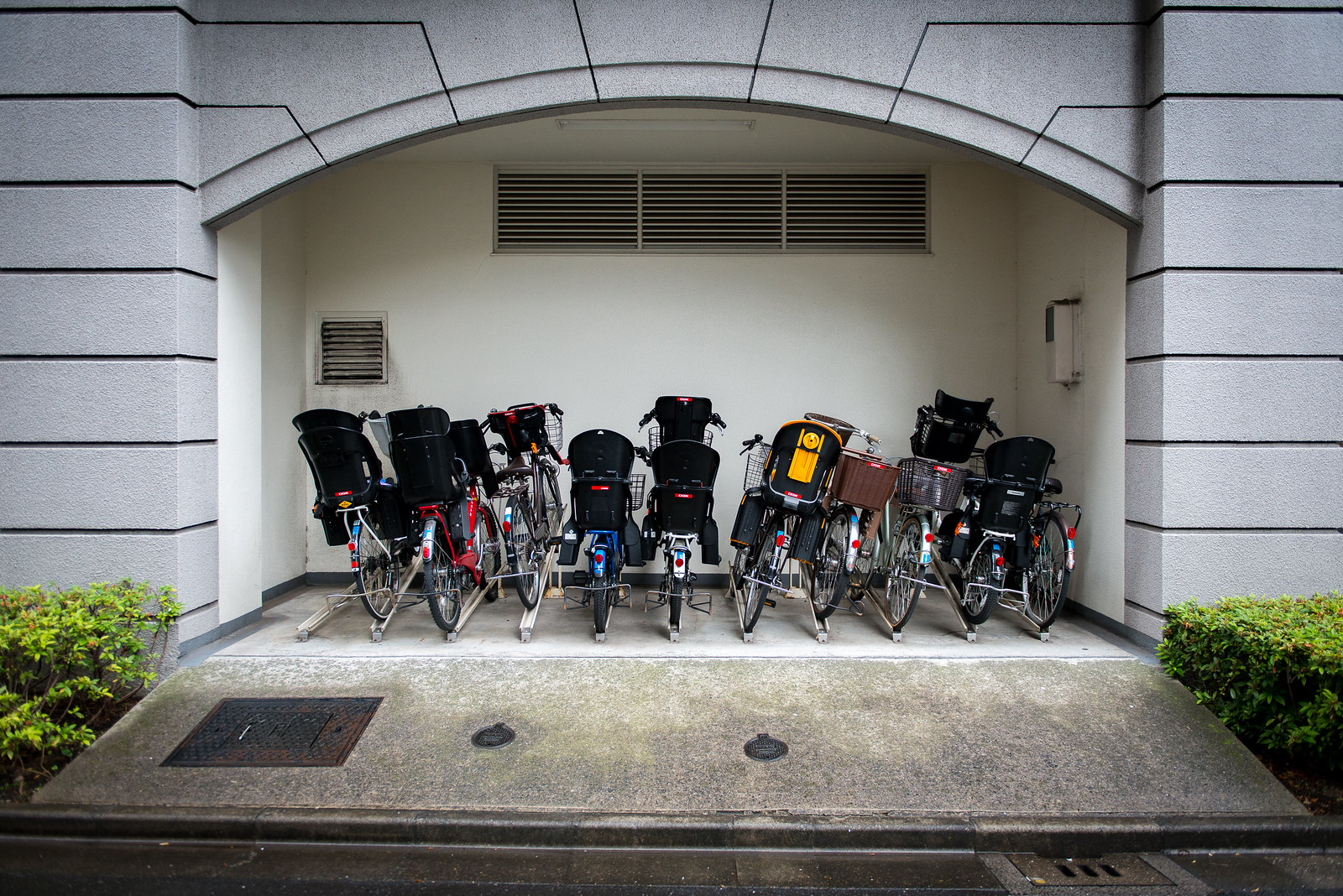This is a photograph of a cluster of bicycles neatly lined up inside a narrow arched overhang attached to a gray stone building. The structure is composed of long rectangular gray stones creating a protective alcove for the bikes. A concrete ramp slopes upwards into the overhang, transitioning from a weathered exterior to a lighter, non-exposed interior floor. The alcove is equipped with several vents for ventilation, including three high up on the back wall and one smaller, lower on the side.

There are ten bicycles in total, mostly rear-facing, with many having distinct features such as child seats and baskets. Specifically, six bikes are equipped with child seats, which are predominately black, and three bikes have baskets attached. The bicycles are secured in a bracket-like apparatus that elevates the front wheel slightly, perhaps for better stability. The bikes display a variety of colors including blue, red, turquoise, white, and black.

Outside the bike parking area, the overhang is flanked by green bushes on either side. A sidewalk with drainage grates runs in front of the alcove, guiding any excess water away. On the wall inside the alcove, there is also a conspicuous white box. This well-thought-out space appears to serve the residents of a nearby apartment building or community facility, particularly those with young children, providing a sheltered spot to park bicycles.